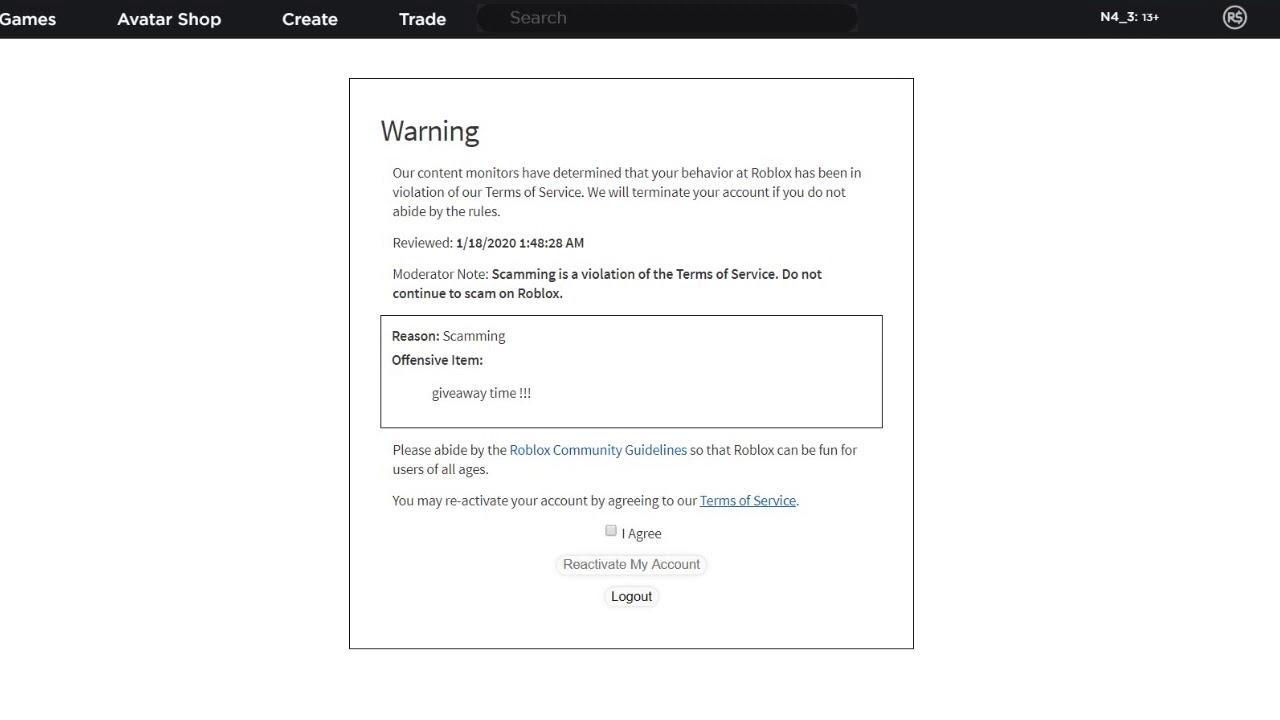The image features a prominent black navigation bar at the top with white text, dividing the screen into several sections: Games, Avatar Shop, Create, Trade, and Search. To the top right of the bar, it displays "N4-3-13+" along with a copyright symbol.

Beneath the navigation bar is a prominent text box containing a warning from Roblox's content moderation team. The warning states: "Our content monitors have determined that your behavior at Roblox has been in violation of our Terms of Service. We will terminate your account if you do not abide by the rules. Reviewed January 18, 2020, 1:48 AM." The moderator's note specifies that "scamming is a violation of the Terms of Service. Do not continue to scam on Roblox." The reason for this warning is listed as "scamming" with the cited offensive item being "giveaway time." 

The message continues by urging the user to follow the Roblox Community Guidelines to ensure a fun experience for all ages. There are instructions indicating that the user may reactivate their account by agreeing to the Terms of Service. Below the message are interactive options, including an "I Agree" checkbox, a "Logout" button, and a "Reactivate My Account" button, providing the user a way to comply with the terms and regain access to their account.